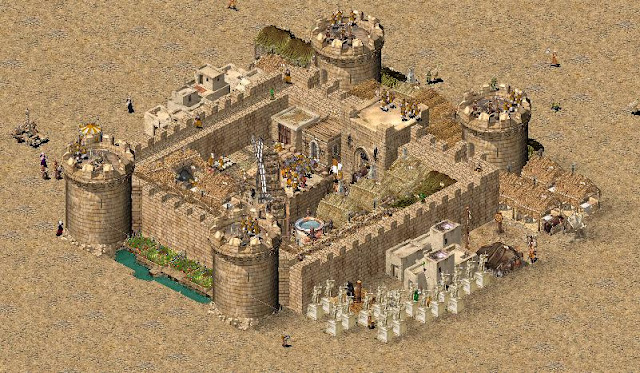This is an illustration resembling a sandcastle with an aerial view of an elaborate, clearly illustrated castle situated in a sandy, almost desert or beach-like environment. The castle is primarily sand-colored and prominently positioned in the center of the image. It features four round towers and a large central courtyard. Scattered throughout the scene, there are multiple people milling about and engaging in activities around the castle. On the right side of the illustration, there are some ambiguous white structures that seem separate from the castle itself. The left side features a vehicle, adding to the scene's bustling atmosphere. Among the sparse greenery, a small patch of water with an unnatural color is visible, enhancing the surreal quality of the image. Various colors, including shades of brown, black, white, blue, green, red, and orange, contribute a rich palette to the scene. The castle and surrounding elements, such as construction materials and additional smaller buildings, suggest that the image might be a computer-generated scene from a video game, offering a stylized and slightly artificial visual experience.